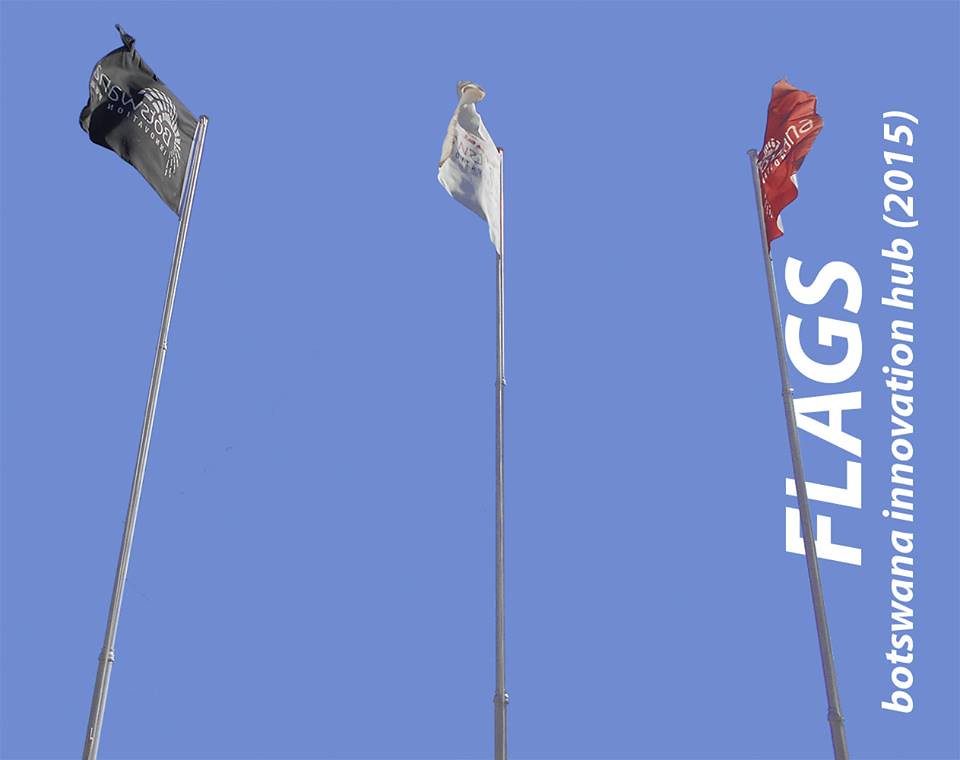The photograph captures a bright, clear blue sky devoid of any clouds, and three high-standing silver metal flagpoles. Each flagpole proudly hoists a flag that flutters in the wind. The left flag is black with white text clearly reading "Botswana Innovation." The middle flag is white, and the right flag is red, though the text on these two flags isn't entirely legible. Despite this, it's likely that all three flags carry similar, if not identical, messages. Along the right edge of the image, there's a watermark-like text oriented vertically that states, "Botswana Innovation Hub 2015" in white font. This scene suggests an event or gathering focused on innovation and entrepreneurship. The photograph is taken from ground-level, emphasizing the tall stature of the flagpoles against the vast, serene sky.